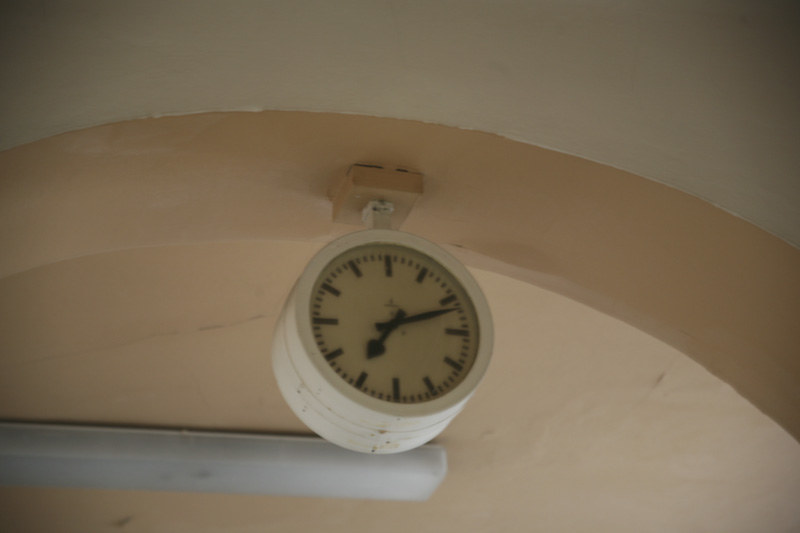The photograph features a small, round analog clock mounted on the ceiling within a pale peach-painted archway. The wall outside the archway is a cream off-white color. This ceiling-mounted clock has a thick white frame and an aged yellow or beige face. The clock face marks the time as approximately 11 minutes past 7 o'clock and lacks numerals, instead having black lines for hours and short dashes for minutes. The hour hand is distinctive with a spade shape at its end, and the minute hand is pointed. A fluorescent light fixture with a cover is also visible behind the clock on the ceiling, though it is not illuminated. The archway itself is painted a dark pink or off-pink color.